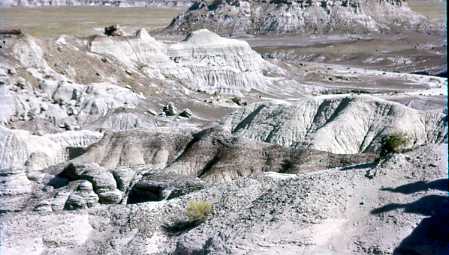The image is a horizontally aligned, smaller-sized rectangular photograph depicting a daytime scene of desert cliffs. The color palette spans gray, green, and brown tones. Dominating the foreground is a flat expanse of dirt accompanied by a single green bush sprouting amidst the barren terrain. In the bottom right corner, shadows—possibly cast by trees or people—add intrigue to the scene. The mid-ground is characterized by a series of low, stratified cliffs with gray tops and brown bands at their base. Ascending from the soil, these rocky outcroppings form a textured but not overly jagged landscape. In the background, a large field of bare soil stretches toward a set of four gray cliffs, adding depth to the composition. The overall atmosphere is earthy and rugged, with a touch of natural greenery breaking the monotony of the rocky surroundings.